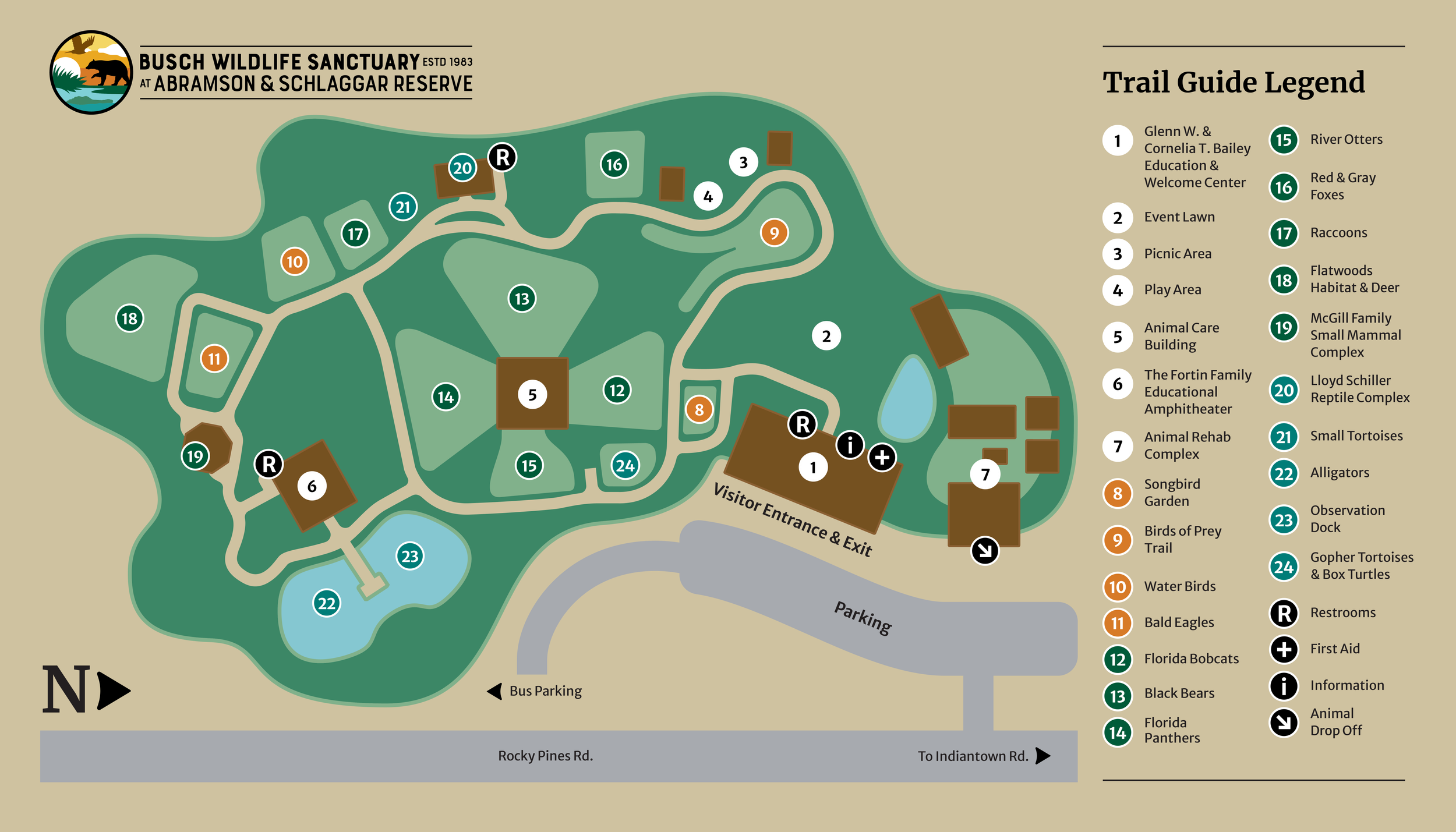This detailed map of the Bush Wildlife Sanctuary at Abramson and Schlager Reserve, identified by their logo of a bald eagle flying over a black bear next to a full moon in the upper left corner, provides a comprehensive overview of the entire grounds. The right side features a Trail Guide Legend, which includes 24 numbered locations indicating key areas such as picnic spots, play areas, different buildings, and animal exhibits, with raccoons in area 17 and alligators in area 22. This legend also marks essential facilities like restrooms, first aid stations, information points, and the animal drop-off area. The map employs a palette of green, light green, brown, and blue to represent various physical features such as buildings, ponds, and water elements, set against a light brown background. Notably, the parking and visitor entrance are explicitly labeled on the map. Rocky Pines Road runs along the bottom, and a directional indicator points north to the right. This detailed and color-coded map ensures that visitors can easily navigate the sanctuary and locate specific areas with ease.